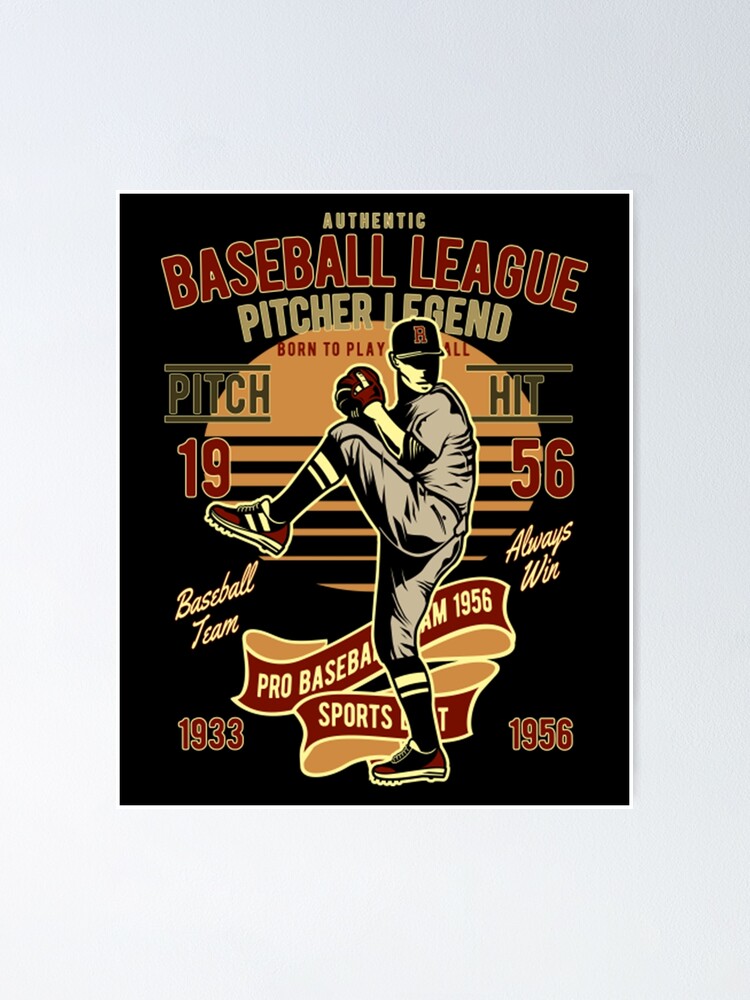The poster features a cartoony-style illustration of a baseball pitcher mid-windup, about to throw a ball. The background is entirely black, enhancing the dramatic effect of the vivid colors in the artwork. At the top center, "Authentic Baseball League Pitcher Legend" is prominently displayed, with "authentic" in small gold lettering, "baseball league" in large red letters stretched almost across the top, and "pitcher legend" in gold.

The pitcher, wearing a Red Sox cap adorned with a red 'B', a gray uniform, black socks with two white stripes, and red cleats with white soles, is depicted in a dynamic high leg kick position. His right hand, gloved, is bent at the elbow and raised near his face, emphasizing his poised, intense stance. 

An orangish sun with black stripes horizontally cutting through halfway serves as a backdrop to the pitcher's figure. Gold lettering, with "pitch 19" written in front of his left side and "hit 56" positioned behind his head, enhances the vintage feel. Additional text scattered around the poster includes "baseball team" beneath his front foot, "always win" near his rear, and a red banner with white and gold trim reading "pro baseball team 1956" behind his leg. The word "sports" in another red banner is partly obscured by his calf. The years "1933" and "1956" are marked in red at the bottom corners, anchoring the poster in historical context. This captivating artwork captures the nostalgia and legend of baseball's golden era.